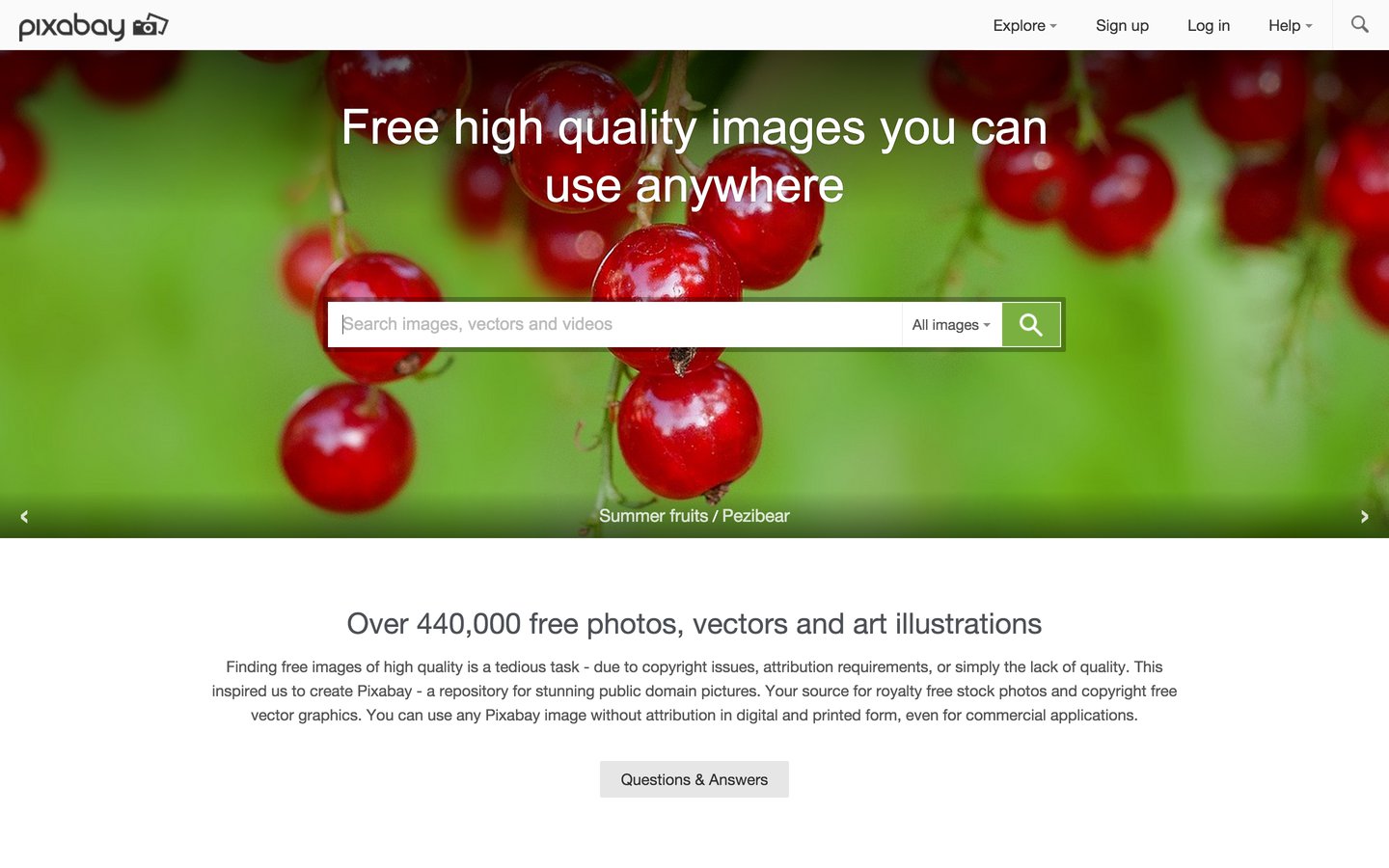Screenshot of a website offering a repository of high-quality, free images, vectors, and videos. At the top, there is a prominent banner with the message: "Free high-quality images you can use anywhere." The name of the website appears to be "Pixarboy." Below the name, options for navigation are displayed, including "Explore," "Sign Up," "Login," and "Help." A search bar is prominently placed with the placeholder text: "Search images, vectors, and videos."

Further down, the website states it offers "over 440,000 free photos, vectors, and art illustrations." A detailed paragraph explains the mission of Pixarboy, emphasizing the challenges of finding free, high-quality images due to copyright issues and attribution requirements. It highlights their commitment to creating a responsible repository of stunning public domain pictures, positioning Pixarboy as a go-to source for royalty-free, copyright-free stock photos.